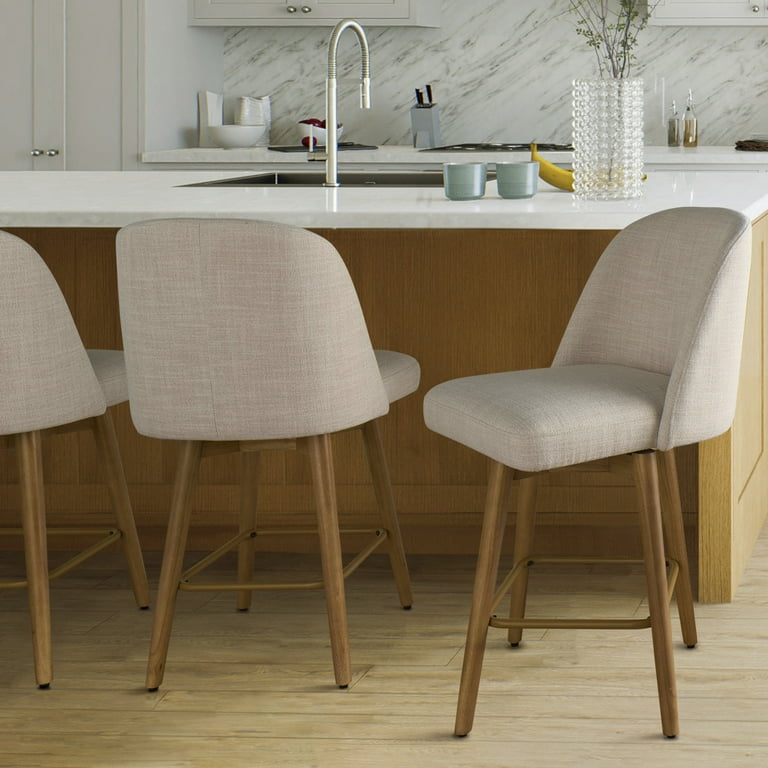The image depicts a modern, well-kept kitchen with a central island featuring a white marble countertop and a sleek white faucet. Centered on the island are two gray coffee cups, a single banana, and a decorative glass vase with intricate designs containing dried flowers or tall plants. The island functions as a breakfast bar, overhanging slightly with space for three barstools. The barstools have off-white or light tan cushions and brown wooden legs, complementing the light wooden floor beneath.

The kitchen is characterized by its bright and clean aesthetic, dominated by white cabinets and a white door presumed to be a pantry. The backsplash consists of elegant white tiles with subtle gray streaks. To the side, additional kitchen elements are visible, such as a stove, a knife block, two bottles likely containing vinegar, and a wooden bowl filled with red apples. The overall ambiance is airy, modern, and meticulously maintained.